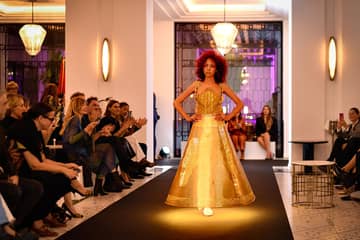In the image, a model confidently struts down a runway, illuminated by a spotlight that creates a golden glow around her and accentuates the brown carpet beneath her. She has shoulder-length, highly textured, reddish-brown hair and light brown skin. Standing with her hands on her hips, she wears a striking golden dress with a corset-like bodice that flares out from the midsection. The setting appears to be an intimate fashion show held in what resembles a ballroom or hotel lobby. The room is sparsely populated, with the audience dressed in shades of black, gray, and white, many of whom are capturing the moment with cell phone cameras. Additional light sources include ceiling-mounted and wall-mounted lights, contributing to the opulent ambiance. To the left of the model, there are a few small tables where more attendees are seated, further enhancing the elegant but private atmosphere. Behind the model, an open doorway or possible two-way mirror reflects even more onlookers, adding depth to the scene.